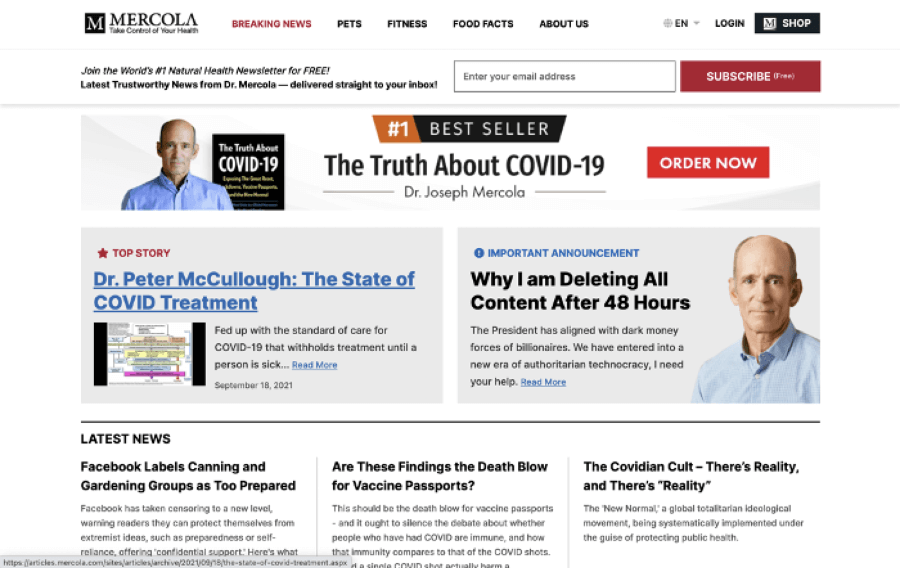Here's a cleaned-up and detailed descriptive caption for the image:

---

This image is a screenshot of a web page from the Mercola website. At the top of the page, a black square with a white 'M' inside marks the logo. Adjacent to the logo, the name "Mercola" is spelled out in black text. Beneath this, a slogan reads, "Take Control of Your Health."

To the right, bold red text displays "Breaking News," and next to it, selectable sections — "Pets," "Fitness," "Food Products," and "About Us" — are highlighted in bold black text. 

Further to the right, an icon of a globe appears, labeled "EN," indicating it as a dropdown menu for selecting language preferences to translate the website. 

At the far right, "Login" is presented in bold black text. Next to "Login," there's a black rectangle containing a white box with a black 'M' inside, followed by the word "Shop" in white text.

On the left-hand side, a promotional message invites users to "Join the world's number one natural health newsletter for free!" It promises the latest trustworthy news from Dr. Mercola delivered straight to your inbox. Below this, a search box with a thin gray border has placeholder text that reads, "Enter your email address." A red clickable button labeled "Subscribe (Free)" in bold white text is beside the search box.

Within this section, there is additional information about COVID-19, featuring an image of a man with gray hair on the sides of his head, wearing a blue shirt. This individual is identified as Dr. Joseph Mercola. 

To the left of this image, a black square contains white text stating, "The Truth About," followed by large bold white text "COVID-19." Adjacent to this, a trapezoid graphic is color-blocked: its larger portion is gray or brown with a bold white number "1," and the smaller black portion reads "Bestseller."

Finally, beneath this graphic, bold black text reiterates "The Truth About COVID-19," identifying the person as Dr. Joseph Mercola.

---